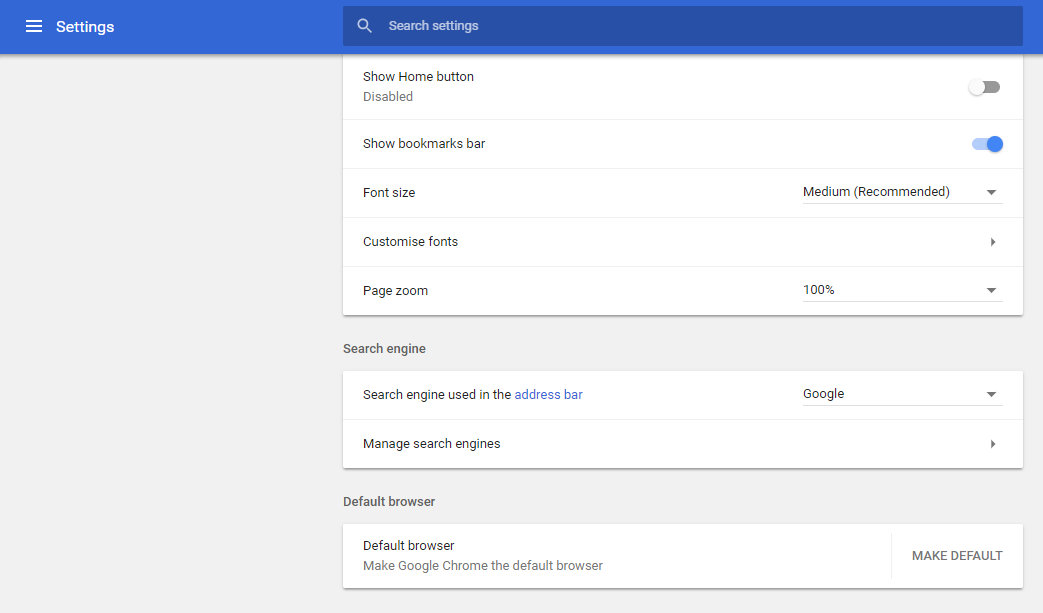This image is a screenshot of a settings menu on a Chromebook. The top of the screen is dominated by a blue bar that prominently displays the word "Settings" on the left. To the right of this bar, there is a darker blue box that functions as a search bar, allowing users to search for specific settings.

Below the blue bar, the screen lists several settings available for customization. These settings include:

- **Show Home Button**: An option that can be toggled on or off to display the home button on the browser.
- **Show Bookmarks Bar**: A setting to either display or hide the bookmarks bar.
- **Font Size**: Allows users to adjust the size of the text displayed on webpages.
- **Customize Fonts**: Provides options to change the style of fonts used.
- **Page Zoom**: Controls the zoom level of webpages.
- **Search Engine**: Gives users the ability to set or change the default search engine.
- **Manage Search Engines**: An option to view and manage the list of search engines available.
- **Default Browser**: Setting to designate the default web browser.

Each of these settings has a corresponding toggle switch or adjustment option on the right side, enabling users to turn features on or off or to customize settings to their preference.